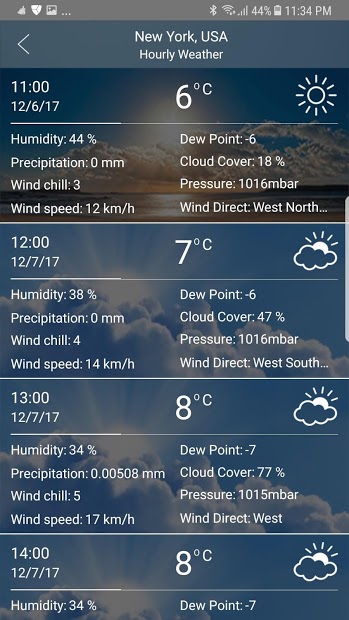The image depicts a smartphone displaying an hourly weather report for New York, USA. The upper part of the screen features a gray border. On the left side of the border, there is a triangular icon divided into three white segments, which appears somewhat unclear. The battery indicator displays 44% in white, and the current time is shown as 11:34 PM. The Wi-Fi reception icon is also white.

The background transitions into a bluish-gray gradient. On the left side of the screen, there's a white arrow pointing left. The text "New York, USA, hourly weather" is clearly visible. 

Below, detailed weather information is listed on the left side:
- At 11:00, on 12/6/17: Humidity is 44%, precipitation is 0 mm, wind chill is 3, and wind speed is 12 KM/H.
- At 12:00, on 12/7/17: Humidity is 38%, precipitation is 0 mm, wind chill is 4, and wind speed is 14 KM/H.
- At 13:00, on 12/7/17: Humidity is 34%, precipitation is 0.00508 mm, wind chill is 5, and wind speed is 17 KM/H.
- At 14:00, on 12/7/17: Humidity is 34%, with temperatures varying as follows: 6°C, 7°C, 8°C, and 8°C.

The screen contains a considerable amount of data, systematically arranged to provide comprehensive hourly weather information.